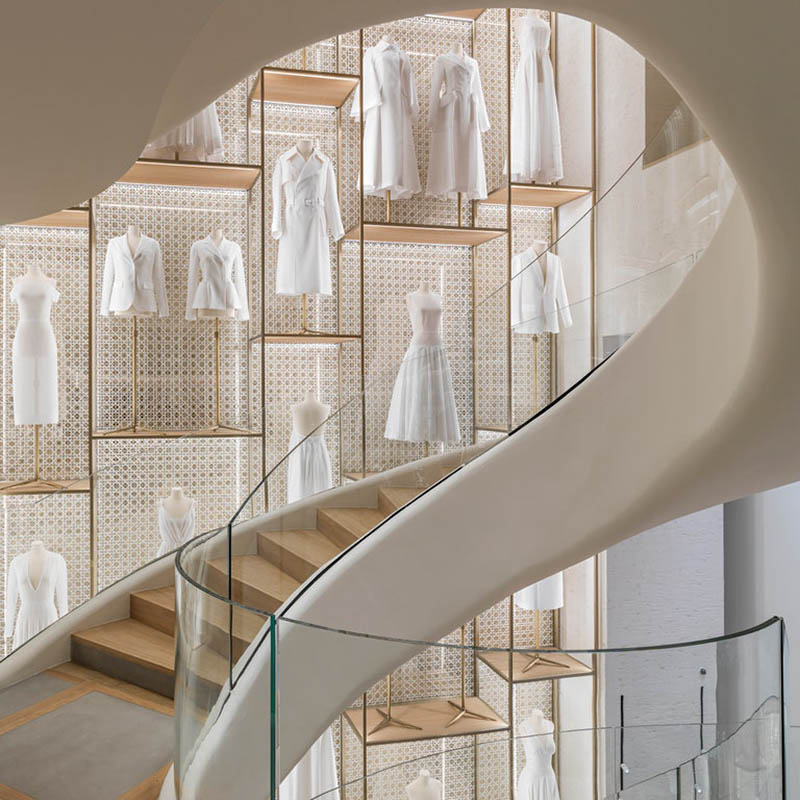The image depicts a modern, high-end store interior centered around an elegant white spiral staircase with smooth sides, ascending from the bottom left to the top left corner. The staircase features light brown wooden steps and a clear, solid plastic railing. The backdrop displays a sophisticated arrangement of medium to dark brown encased rectangles, trimmed in gold, spanning from the floor to the ceiling. Within these rectangles, a variety of white garments—including dresses, blazers, shirts, and coats—are meticulously showcased on gold mannequins with heads and legs omitted, emphasizing the clothing. The overall scene exudes a luxurious and high-tech ambiance, giving a glimpse of an artistic and functional space where the staircase serves as both a pathway and a visual focal point amidst the elegant display of fashion.